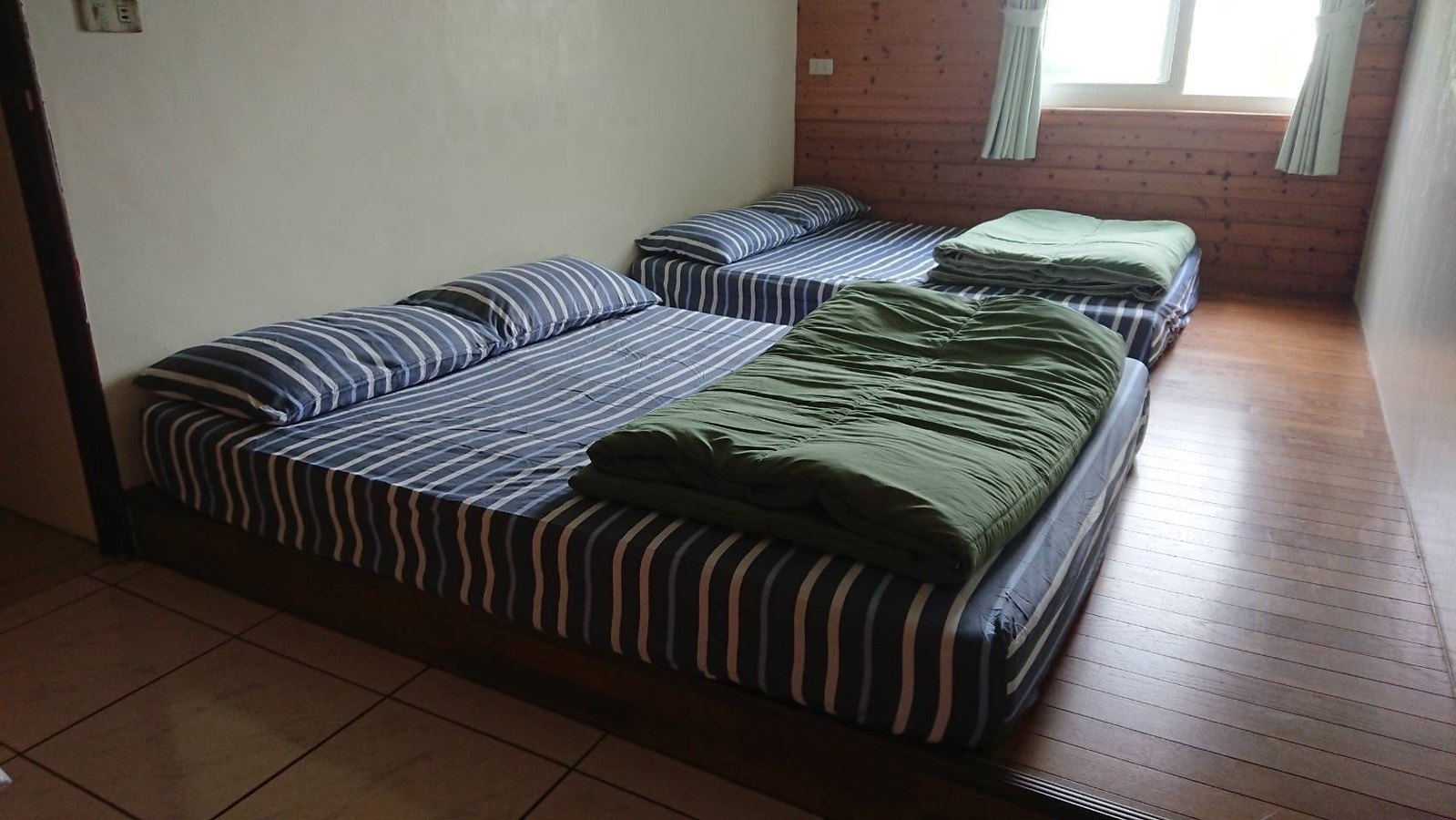The image depicts a narrow, rectangular bedroom, possibly a hotel room, with two king-size beds placed side by side against a cream-colored wall. The room features a wooden floor with dark wood planks running from the right side to the left. Adjacent to this is a raised area that transitions into a tiled section with large, grey, rectangular tiles. 

The beds are directly on the floor, covered in bedspreads with alternating light blue, dark blue, and cream stripes. The pillows match the bedspreads but have stripes running in the opposite direction. Each bed has a green blanket folded at the foot; the closer bed has a dark green blanket, while the one nearer to the window has a lighter green blanket. 

On the wall to the left, which continues in the same direction as the floor planks, there is a window fitted with white curtains. A bit of the cream-colored wall is visible to the right of the window. Behind the beds, on the left side of the photo, there's a brown door with black trim. This detailed setting suggests a cozy and functional space, blending rustic and contemporary elements.